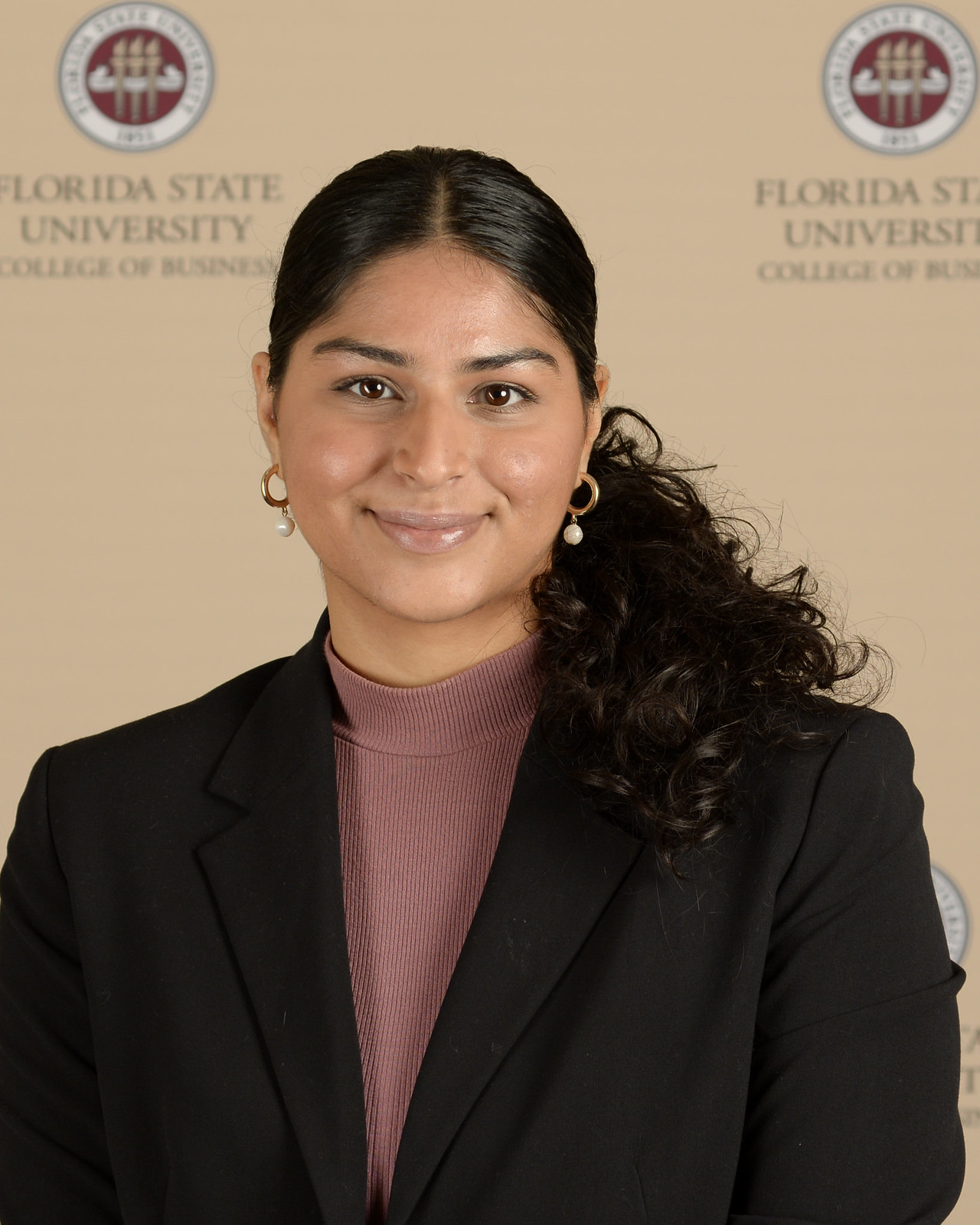A tall rectangular photograph features a young woman standing in front of an advertising sign for Florida State University College of Business. She is centered in the image and visible from the chest up, her shoulders occupying most of the frame. The backdrop is a beige-colored wall with a burgundy circular logo featuring three torches and a silver outer ring that repeatedly reads “Florida State University College of Business.”

The woman has light brown skin and is wearing a black blazer over an almost turtleneck, beige-pinkish gray knit shirt. Her dark brown curly hair is slicked back and cascades in a ponytail over her right shoulder. She has brown eyes, black eyebrows, and is adorned with gold hoop earrings with pearls dangling from them. She is smiling, wearing pink lip gloss, and her relaxed posture radiates confidence and warmth. The detailed backdrop and her attire give the impression of a professional and poised appearance.